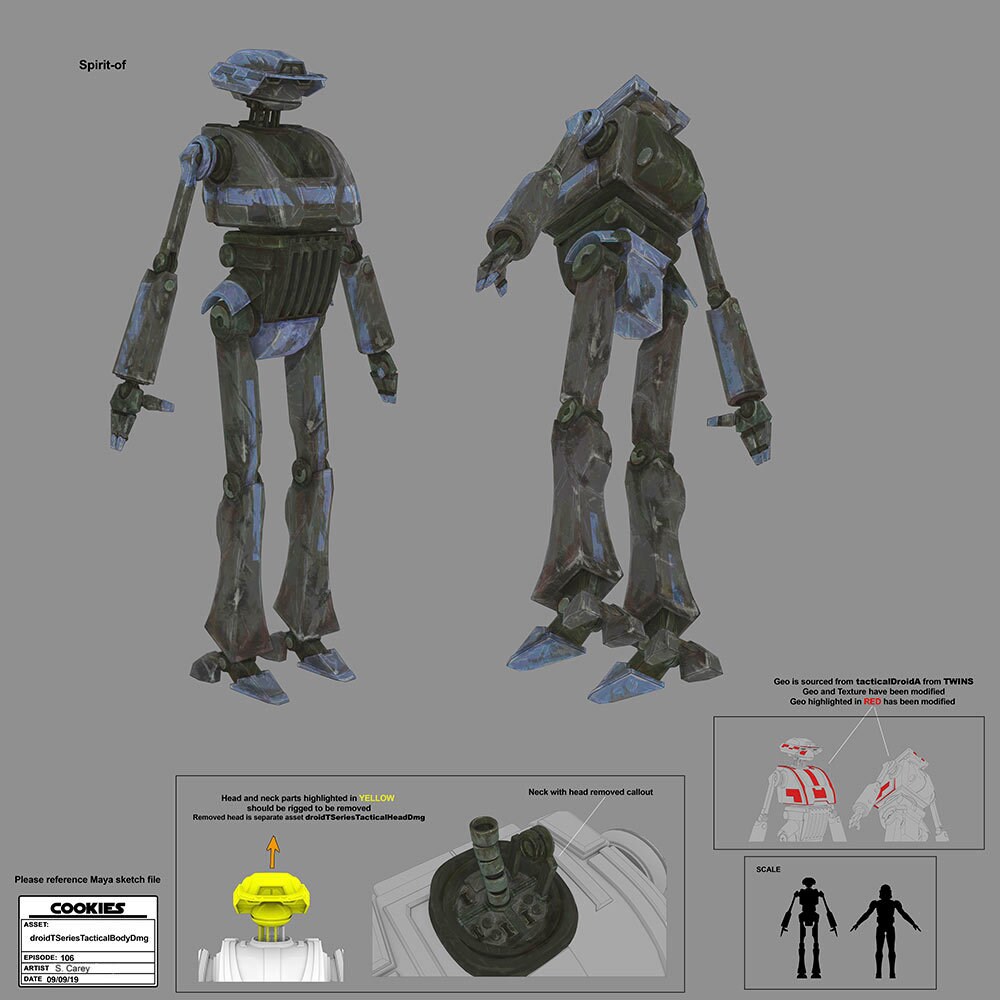This detailed diagram depicts two silver, mechanical-looking T-Series tactical droids, showcasing both their full bodies and specific parts with instructions. In the top left corner, the phrase "spirit-of" is written in black. The bottom left advises to "please reference Maya's sketch file." In a layout resembling nutrition facts, there’s text listing various details: "cookies, asset, droid T-Series, tactical body DMG, episode 106, artist S. Carry, date 09-09-19."

The main section includes a detailed illustration of head and neck parts highlighted in yellow, indicating that "the head should be rigged to be removed," and an additional note that the "removed head is a separate asset." The rectangle caption elaborates: "droid T-Series, tactical head DMG," accompanied by an image of the head depicted in yellow below. To the right, text clarifies "neck with head removed callout," showing a dissected view of the neck in black.

Another callout explains that the "geo is sourced from tactical droid A from twins," noting that "geo and texture have been modified," with red highlights indicating the modified sections. 

The droids are skinny, faceless, and mostly gray. One stands sideways while the other appears to be tipping over from the back. At the bottom, various smaller windows provide further annotations and visual details, including the structural diagrams and silhouettes of the robots, with some parts painted red.